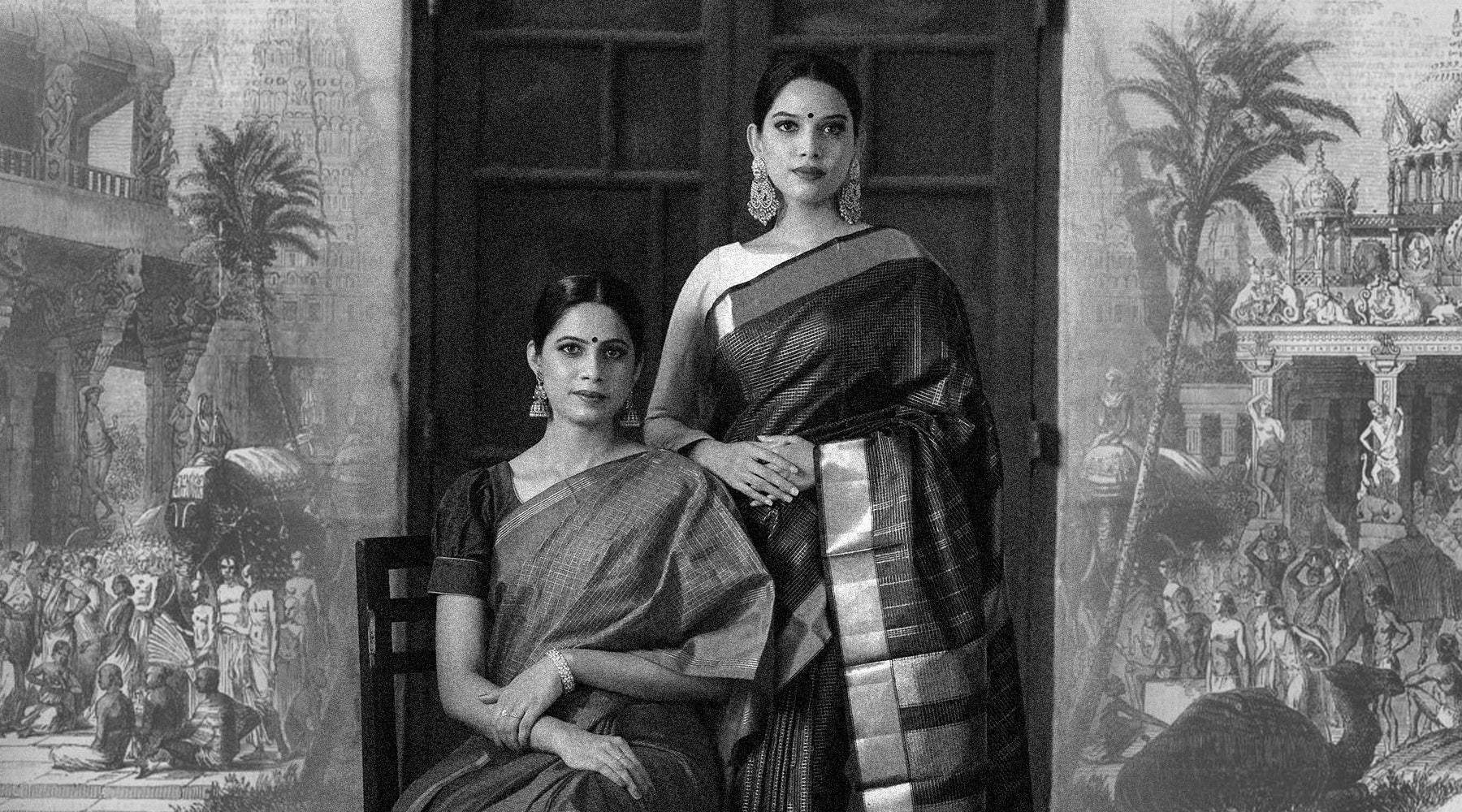This black-and-white photograph captures two Indian women standing in front of a large wooden cabinet. The seated woman is on a sideways turned wooden chair, while the standing woman rests her arm over the other’s shoulder. Both women are adorned in traditional Indian attire, featuring shawls that stretch across their chests and flow into long dresses. They have their black hair parted in the middle, slicked back, and tied up. Each wears dangling, elaborate moon-shaped earrings and a bindi dot on their forehead. Their hands are clasped in front of them. Behind the women, the image reveals an intricate illustration of a bustling village scene. This vivid backdrop features ancient two-story buildings, crowded streets with people, wagons, and figures carrying items on their heads, as well as palm trees, contributing to the lively ambiance.